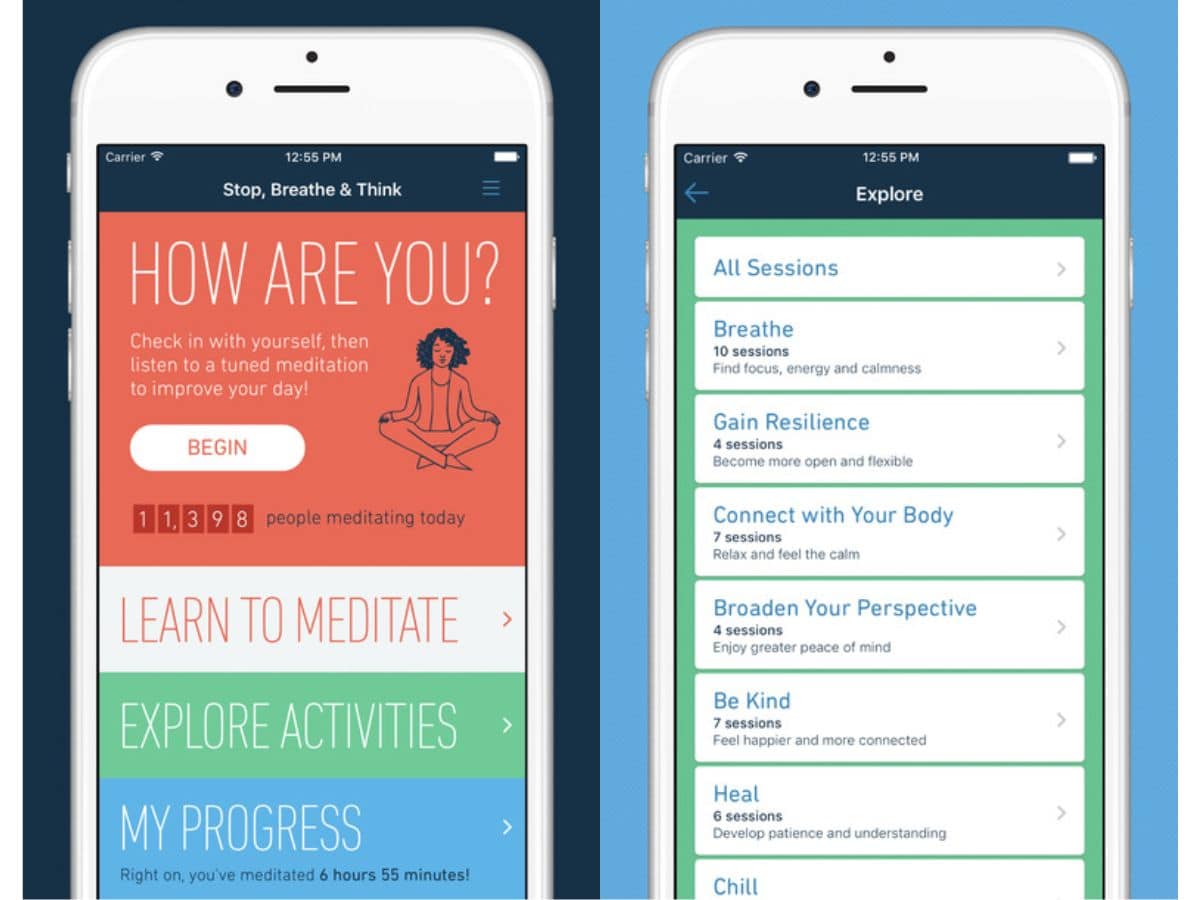The image consists of two pages depicting a phone interface with comprehensive and detailed features.

**Left Page:**
- The phone's screen is encased within a white body with visible bezels and side buttons.
- At the top of the screen, there's a blue header displaying "Stop, Breathe & Think" along with the time, carrier information, and battery status.
- Below the header, an orange section contains white text stating, "How are you? Check in with yourself and listen to a meditation to improve your day."
- Further down is a prominent white button labeled "Begin" next to a small illustration of a woman sitting cross-legged with her eyes closed, symbolizing meditation.
- Beneath the illustration, there is a statement: "11,398 people meditating today."
- At the bottom, a white section reads "Learn to Meditate," followed by a green section labeled "Explore Activities."
- A blue section at the bottom lists the user's progress: "Right on! You've meditated 6 hours and 55 minutes."

**Right Page:**
- The header reads "Explore" in blue.
- Below are multiple white boxes with blue text, each representing a different meditation category and the number of available sessions:
  1. All Sessions
  2. Breathe
  3. Gain Resilience
  4. Connect with Your Body
  5. Broaden Your Perspective
  6. Be Kind
  7. Heal
  8. Chill
- Each category box includes a brief description of its focus or objective.

This detailed caption captures the essence and functionality of the phone interface designed to guide users through their daily meditation practices.